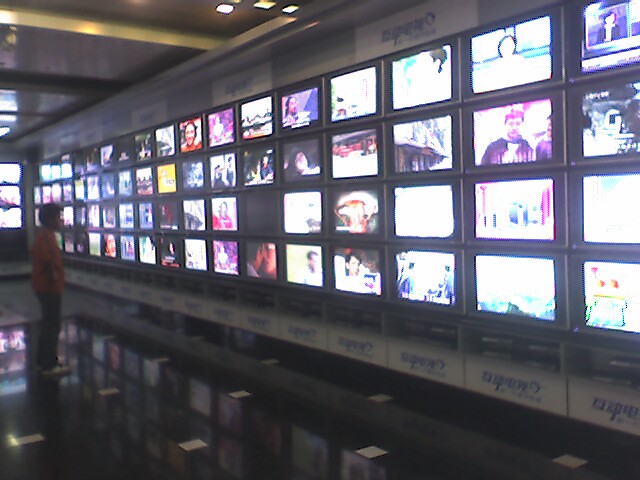The image depicts a dimly lit, expansive room dominated by a vast wall of television screens neatly stacked in a grid four rows high and extending approximately 17 columns wide across the room. The screens, possibly measuring around three feet by two feet, each display varied content, suggesting a mix of channels, images, and possible media types such as movies, TV shows, or documentaries. The wall of screens curves slightly to the left at the far end, continuing the array and adding to the magnitude of the display.

Standing on the highly reflective, black polished tile floor with small white tiles periodically aligned in a grid pattern, a lone individual can be seen observing the screens. The person, likely a man, is dressed in a short-sleeved orange shirt, dark pants, and white sneakers, and has a short haircut. Below the screens, text is visible but unreadable, potentially flipped upside down. The ceiling features some illumination and gold fixtures that faintly light the room, highlighting a sleek steel or aluminum frame supporting the screens. The overall atmosphere resembles a control room or a technologically advanced surveillance space.